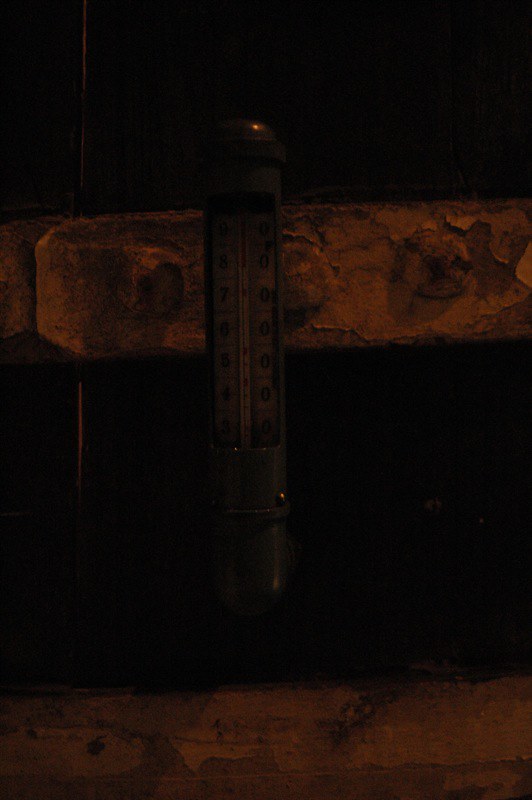In this hauntingly atmospheric, vertically-oriented color photograph taken in the dark, the focal point is an old metal gauge, positioned precisely at the center of the composition. The photograph's low lighting renders most of the image jet black, emphasizing the mysterious aura of the scene. The gauge, likely an antique, is gray and features a cylindrical center secured with visible screws. Its top is rounded, and the gauge displays a numerical scale: on the left side, numbers range from 3 to 9, reminiscent of a thermometer, while the right side contains a series of zeros progressing upwards in the center section. 

Faint lines between the numbers enhance the intricacy of the device. The gauge is mounted on a wall, its paint peeling away dramatically, revealing shades of deep orange that evoke the warm, flickering light of a distant fire, giving the image an antique sepia tone. Below the gauge, another section of the wall similarly shows layers of peeling paint. The dark, undefined background amplifies the contrast, making the illuminated portions of the gauge and wall appear as though steeped in history, captured perhaps in the glow of an old fireplace.